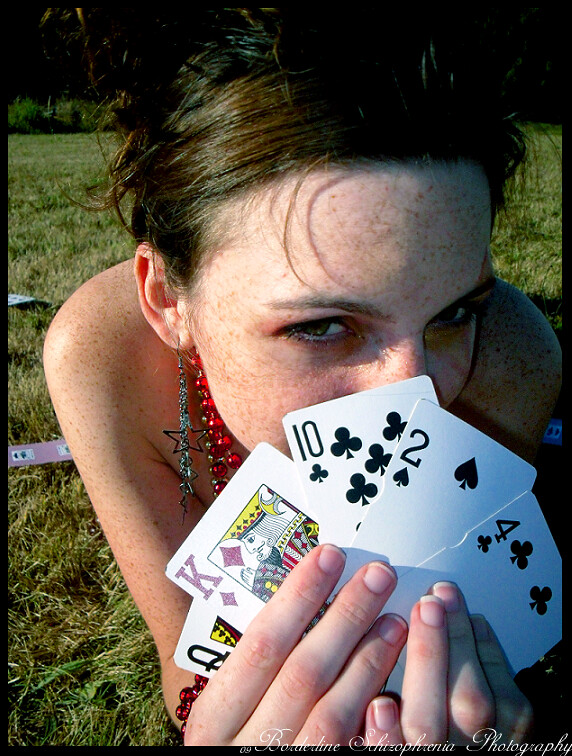In this vibrant outdoor scene, a lush green field stretches out under a sunny sky, with a small hedge forming a verdant backdrop. On the ground, several small white and red objects with black numbers lie scattered. At the center of the image, a young girl with reddish-brown hair and a profusion of freckles stands, her face slightly pink from the sun. She appears playful and slightly mischievous as she partially conceals her face behind a fan of five playing cards. The cards she holds include the four of clubs, the two of spades, the ten of clubs, the king of diamonds, and a queen from one of the black suits, although it’s unclear whether it’s the queen of clubs or spades. The girl, dressed in a sleeveless outfit reminiscent of a swimsuit and adorned with beads, adds a touch of youthful exuberance to the serene setting.